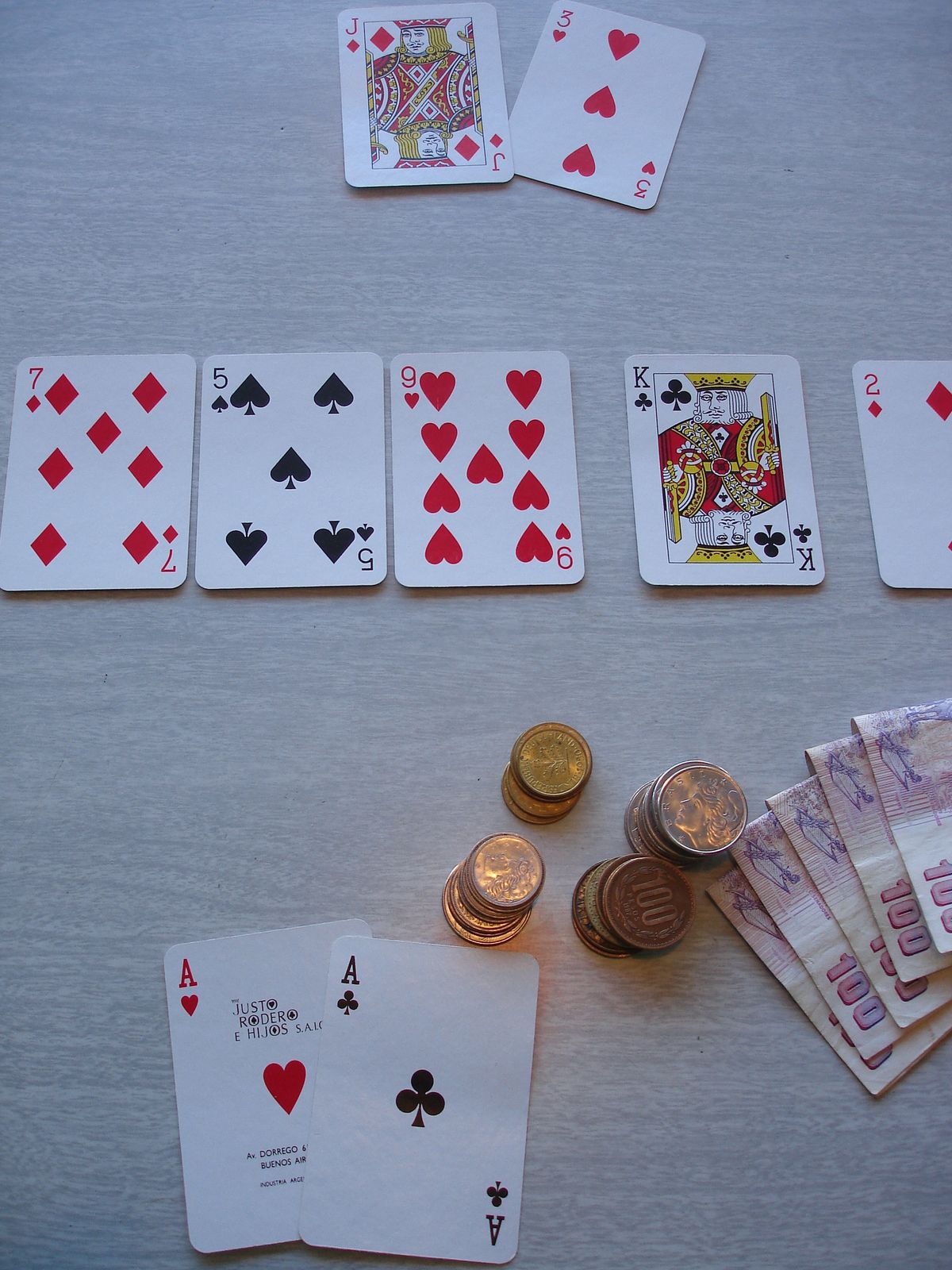The photograph captures a tense moment in a Texas Hold'em poker game. At the center of the rustic table, five community cards are fanned out, showing a seven of diamonds, five of spades, nine of hearts, king of clubs, and just peeking out from the right edge, a two of diamonds. On the opposite end of the table, two cards are laid face-up: a jack of diamonds and a three of hearts. Closer to the camera, another set of two cards lies prominently displayed – an ace of hearts paired with an ace of clubs, suggesting a strong hand. In front of these aces, four neat stacks of coins and four folded bills, peach and white in color with a ruby-tinted '100' emblazoned on them, hint at a high-stakes game. The currency appears to be Eastern European, adding an exotic element to the setting. The overall composition draws the eye into the action, hinting at the intensity of the moment and the strategic decisions in play.